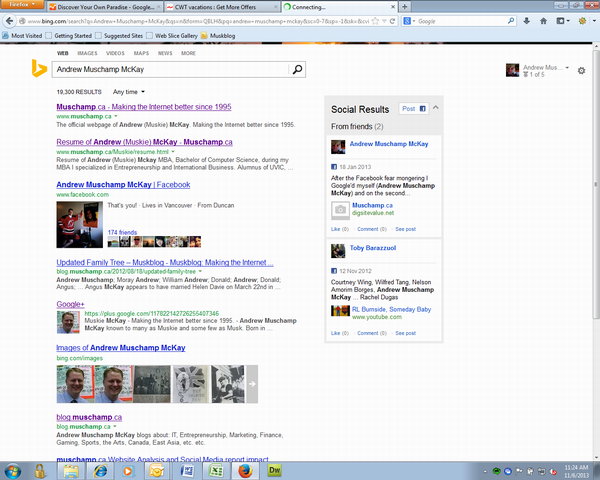The screenshot captures a Bing search result page dated around the early 2000s, as indicated by the vintage appearance of the Windows operating system interface. The top browser bar shows multiple open tabs, including "Firefox," "Set up your own paradise," "Google," "CWT vacations," and "Get more offers." The active tab is labeled "connecting."

In the main content area, the search query is for "Andrew Mushkamp McKay." The search results prominently display links such as "Mushkamp.ca," which declares, "Making the internet better since 1995," and a resume titled "Resume of Andrew Musky McKay." Additional links listed include his profile on Facebook, family tree updates, and entries from the "Mushk blog," alongside results for Google Plus and images related to Andrew Mushkamp McKay. At the bottom of the search listing, there is a final entry leading to "blog.mushkampmckay."

On the right side of the search results page, there is a section marked "social results from friends." This portion highlights two individuals: Andrew Mushkamp McKay and Toby Barizmali, suggesting connections or interactions with the searcher. Further right, there is a truncated text, "Andrew Musk... 105," implying another potential search result or option.

The bottom bar of the screen features the traditional Windows menu indicative of earlier Windows versions, further dating the screenshot to the early 2000s digital environment.